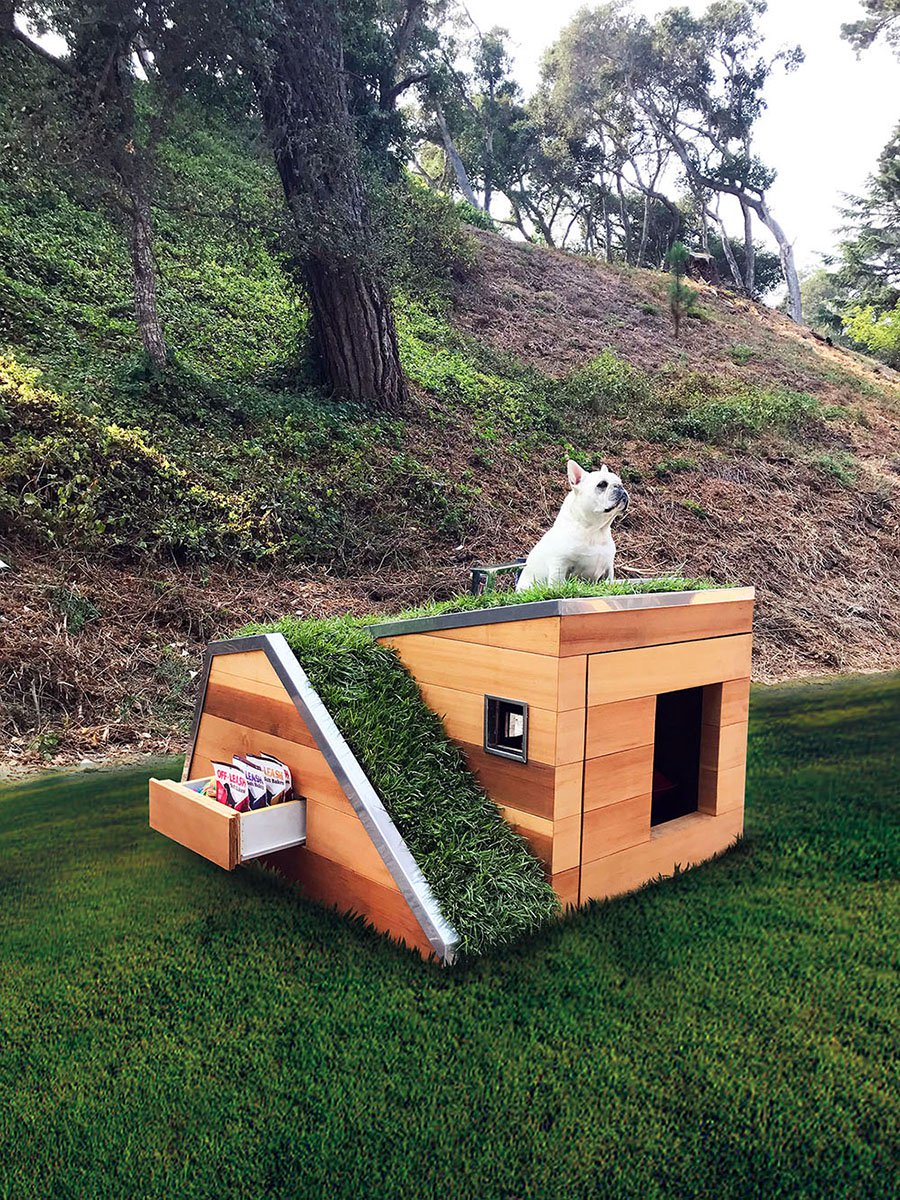In this photograph, a small white pug is perched atop a very fancy, new wooden doghouse. The doghouse has a unique design featuring a ramp covered in lush green grass leading up to the grassy roof, where the dog sits contentedly. Below, the doghouse has a doorway and a small window that add to its charm. On the left side, an open drawer reveals what appears to be dog treats. The entire scene is set on a meticulously manicured lawn, with a picturesque hill and a few trees in the background, under a clear, blue sky.